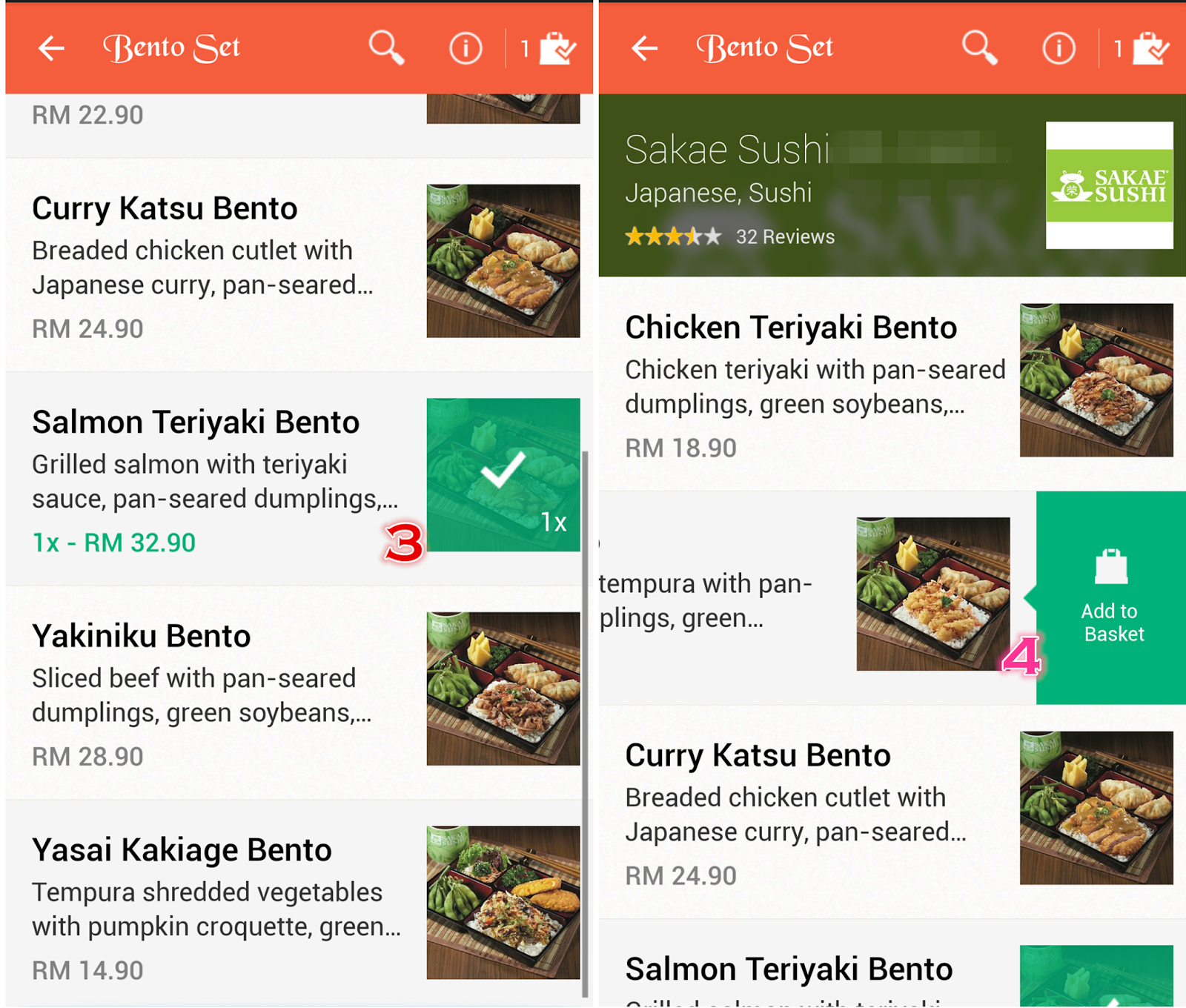This image captures the digital menu of a restaurant called Sake Sushi, displayed on a mobile device. The menu reveals a variety of Japanese cuisine offerings, prominently featuring bento sets on pages 3 and 4. Diners can explore an array of dishes, including curry katsu, teriyaki, and yakiniku, each accompanied by detailed descriptions and enticing photographs. The prices are listed in RM—a currency not immediately familiar, yet signaling a location-specific touch.

Boasting 32 reviews and an impressive 4.5-star rating, Sake Sushi presents itself as a tempting option for anyone seeking Japanese culinary delights. The visuals suggest appetizing and beautifully presented meals, further enhancing the appeal of dining here. The restaurant's diverse menu features not only teriyaki and katsu dishes but also an implied selection of sushi, making it a well-rounded establishment for Japanese food enthusiasts.